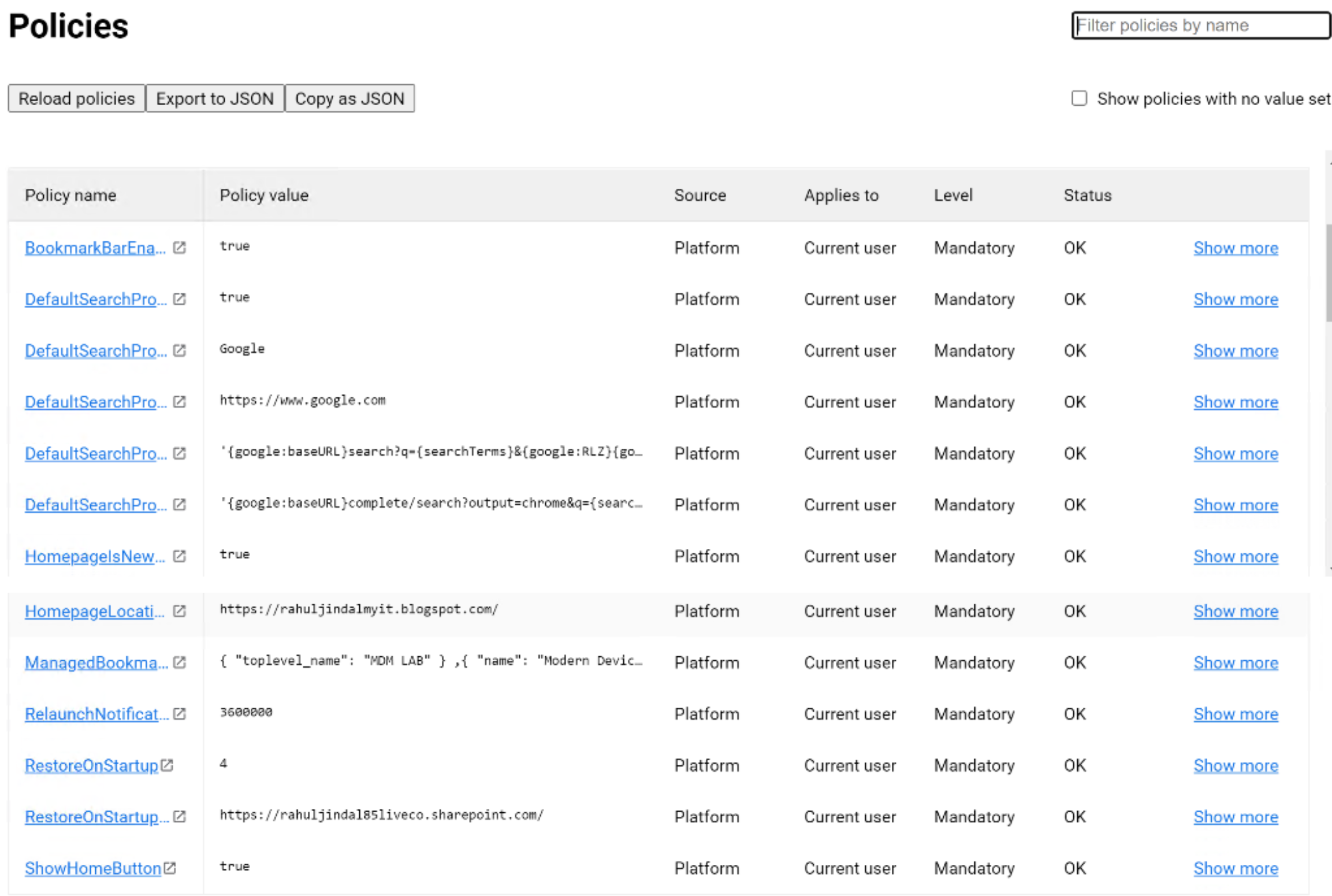The webpage titled "Policies" features a bold black heading, set against a white background. On the same horizontal line as the "Policies" heading, there is a search bar located on the right side. The search bar contains the text "Filter policies by name." Next to the search bar, there are three distinct tabs: "Reload Policies," "Export to JSON," and "Copy as JSON."

Below these elements lies a comprehensive table with grey-colored headings. The columns in the table are labeled as follows: "Policy Name," "Policy Value," "Source," "Applies To," "Level," and "Status." 

In the "Policy Name" column, each policy name is displayed in an underlined blue font, suggesting they are clickable links. Example policy names include "Bookmark Bar ENA" and "Default Search Pro," among others. 

The "Policy Value" column contains entries such as "True" and "Google," all rendered in black font. The table continues with similar structured data, providing a meticulous organization of policy information for users.